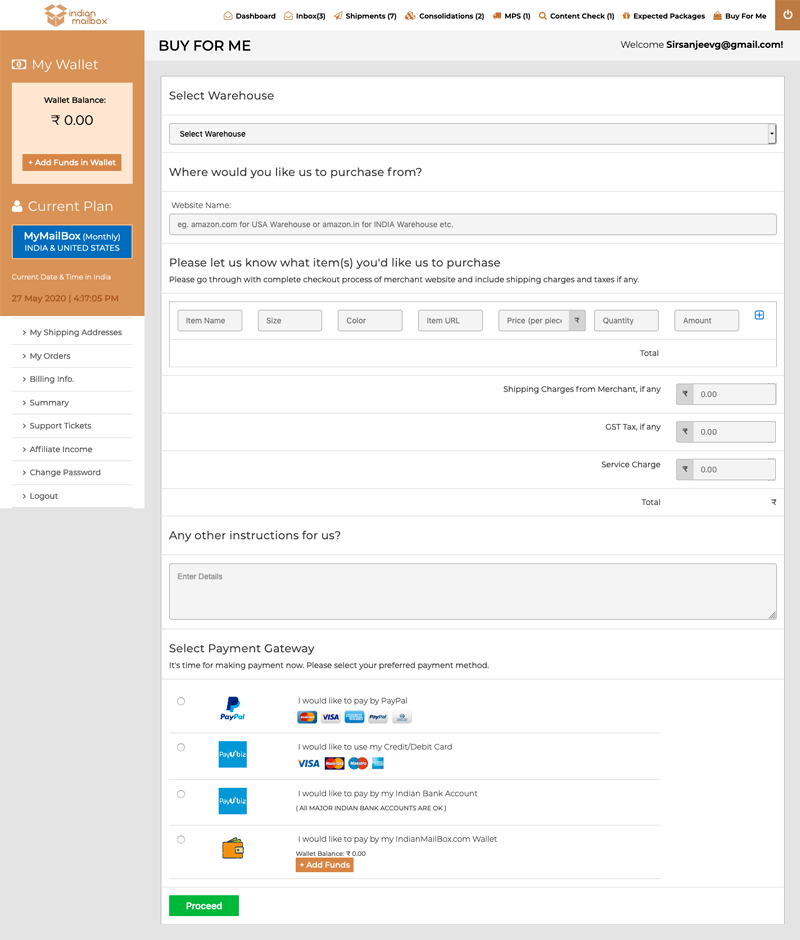At the top of the page, the background is white with the title "Indian Mailbox" prominently displayed in an orange color. Just below, an open box icon, matching the same orange hue, is depicted. In black text, the following categories are listed: "Dashboard," "Inbox (3)," "Shipments (7)," "Consolidation (2)," "NPS (1)," "Content Check (1)," "Expected Packages," and "Buy for Me."

On the left-hand side, there is an orange rectangle labeled "My Wallet." Within it, a lighter square contains black text reading "My Balance," followed by "0.00" in black, although the currency is unspecified. Another orange rectangle within this section features a white plus sign and the words "Add Funds to Wallet." Beneath this, in white text, it says "Current Plan."

Next to the current plan, there is a blue rectangle with white text reading "My Mailbox Currency," indicating the usage of both "Monthly India" and "United States." Displayed in white text are the current date and time in India, presented as "27 May 2020" in a burnt orange color, alongside "4:17:05 PM."

A white rectangle further down lists various options in black text: "My Shipping Address," "My Orders," "Billing Info," "Summary," "Support Tickets," "Affiliate Income," "Change Password," and "Logout." Another black text label reads "Buy for Me."

This section prompts users to select a warehouse, asking, "Where would you like us to purchase from?" The options include "Amazon.com for the US Warehouse" and "Amazon.in for the India Warehouse," requesting users to specify their desired items for purchase.